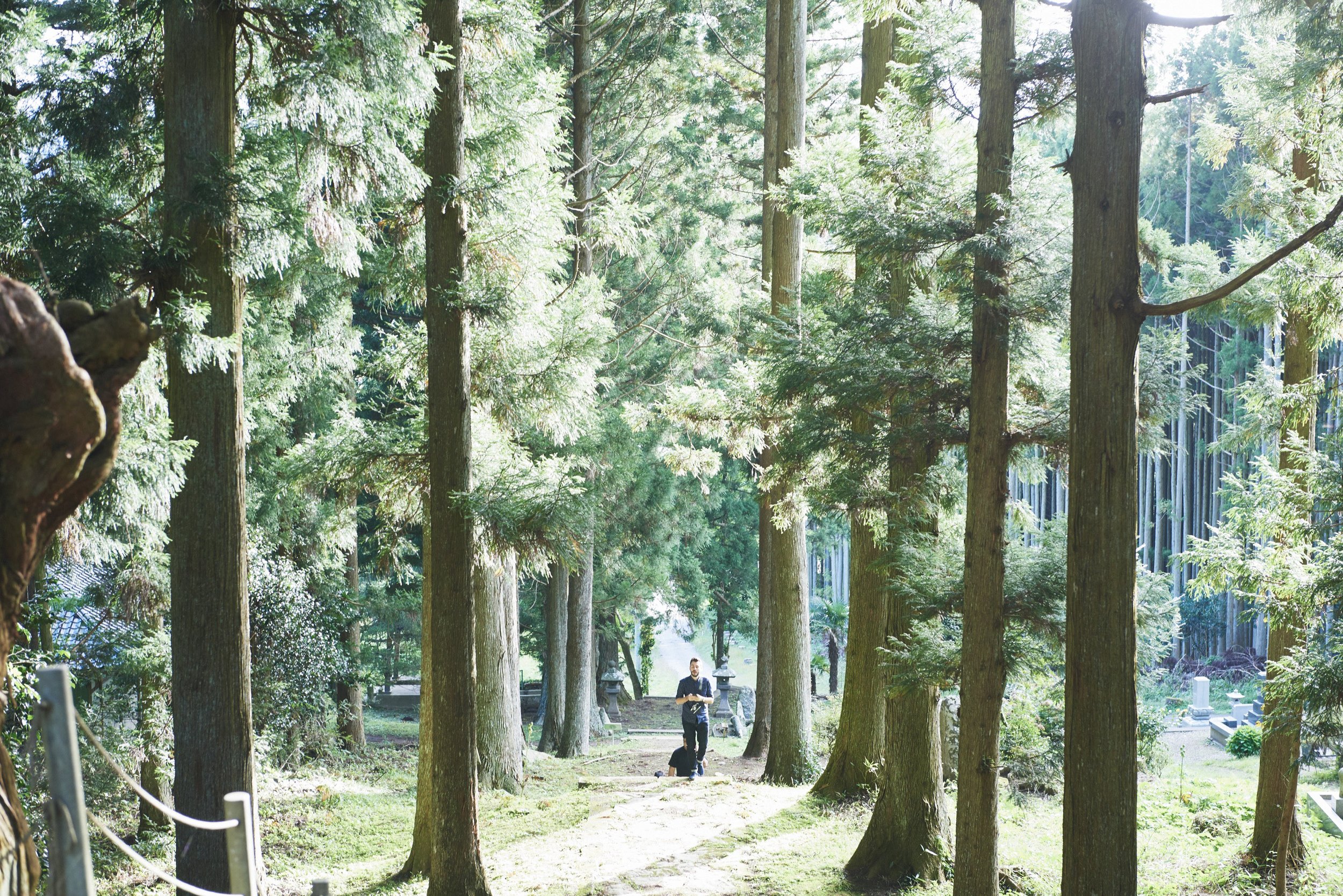The image depicts a vibrant forest scene with towering trees, possibly resembling giant redwoods due to their impressive height. Their greenish-brown bark stands out amidst the scenery. Dark gray lines reminiscent of tree trunks dominate the upper part of the image, interspersed with white and green foliage that appears almost feathery and scattered randomly. The ground beneath is stark white, contrasting sharply with the dense, textured canopy above.

In the foreground, a man dressed in dark clothing stands on a path that meanders through the forest, providing a sense of scale; he appears significantly smaller than the massive tree trunks that stretch far beyond the visible frame. Another figure is visible in the background, slightly elevated, suggesting they are walking down a slope or path. Decorative pillars flank the trail in the distance, adding an architectural element to the natural landscape. There's a hint of lighter gray trees further back, with indistinct structures that might be gravestones, adding an air of mystery to the scene. 

Additionally, in the bottom left corner, a brown structure with a white line on top — possibly ropes or steps — indicates that the image might have been taken from an elevated position. The overall atmosphere showcases the forest’s grandeur and the serene trail winding through it, under the broad daylight.